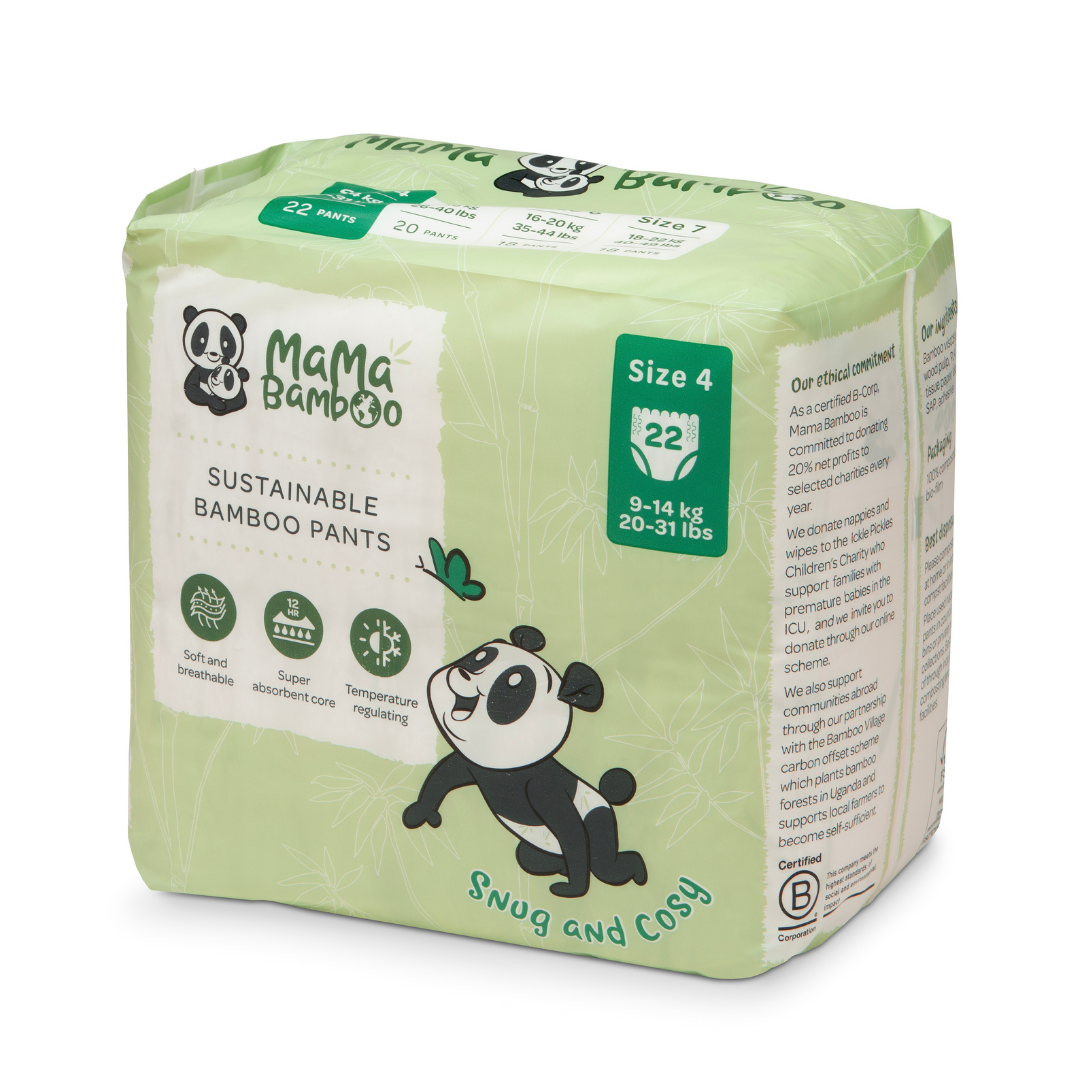The photograph displays a pastel green bag of baby diapers adorned with light white stencils of bamboo plants. On the bottom right of the package, a playful cartoon panda character is depicted, accompanied by a smaller illustration of a panda wearing a diaper. Below this charming depiction, green, childlike text declares the diapers "snug and cozy." The packaging indicates it contains size 4 diapers in a forest green rectangle on the top right corner, detailing that the pack includes 22 units, suitable for babies weighing 9 to 14 kilograms (20 to 31 pounds).

The top left section of the bag features a rough-edged white outline with a white background, showcasing an illustration of a larger panda cradling a baby panda. Adjacent to this, the brand name "Mama Bamboo" is printed in green text with an earth symbol cleverly incorporated into the second 'O'. Beneath this, black text reads "Sustainable Bamboo Pants."

Three green circles at the bottom middle of the package highlight the key features of the diapers: "soft and breathable" with an icon of three white layers and arrows; "12-hour super absorbent core" denoted by five water drops beneath a white surface; and "temperature regulating" symbolized by a combined sun and snowflake graphic.